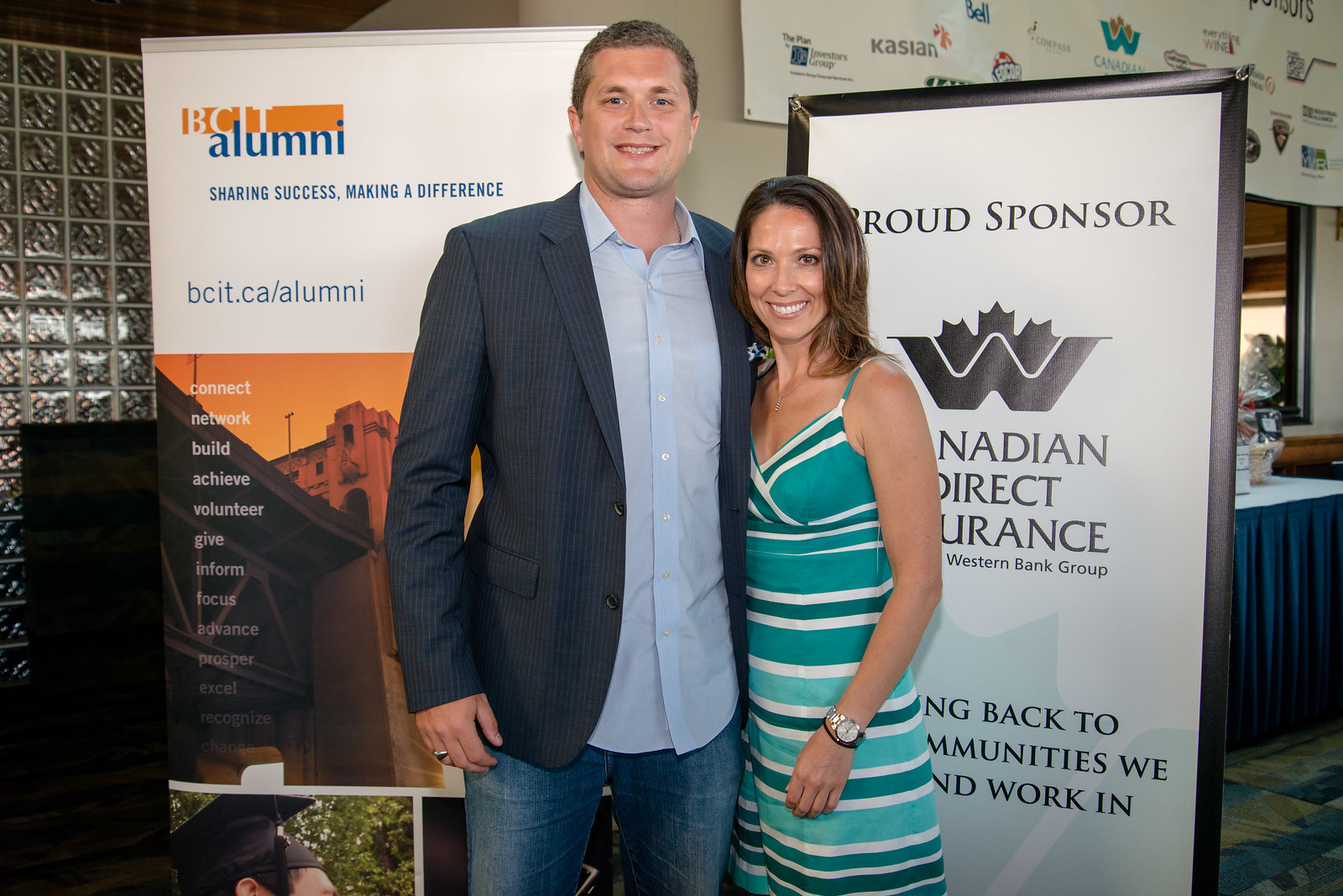In the image, a man and a woman are standing side by side, looking directly at the camera. The man, positioned on the left, is Caucasian with short blond hair, and appears to be in his early 30s. He is dressed in a blue suit jacket layered over a light blue dress shirt, which is untucked, and paired with blue jeans. To his left, on the right side of the image, is a Caucasian woman with shoulder-length brown hair, wearing an aqua and white striped dress.

They are posed in front of two prominent signs. The sign on the left is for BCIT Alumni and features the text "Sharing Success, Making a Difference" at the top, followed by a URL "bcit.ca/alumni". This sign also lists motivational words such as "Connect, Network, Build, Achieve, Volunteer, Give, Inform, Focus, Advance, Prosper, Excel, Recognize". Beneath the text, there is an image of a building set against an orange sky. The sign on the right, partially obstructed by the woman, reads "Proud Sponsor" and includes a logo resembling a fancy 'W.' It mentions "Canadian Direct Insurance" and "Preston Bank Group" as sponsors. The overall setting is bright and clear, indicative of good lighting.